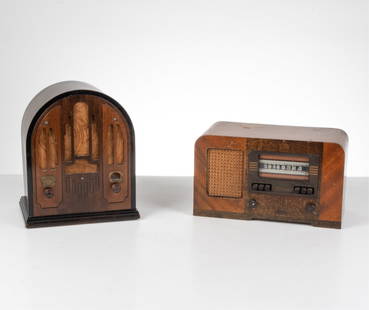This photograph features two vintage radios displayed side-by-side on a white surface with a white background. The radio on the left is styled like an arched doorway or cathedral, characterized by a curved top and flat bottom. It's predominantly dark brown with some lighter brown accents on the front. The radio’s exterior showcases intricate woodwork, albeit slightly blurry. It features a knob on both the right and left sides and sits on a darker, thin base. 

The radio on the right has a rectangular shape with slightly curved top corners, finished in lighter brown wood. This radio includes a central white strip with black numeric markings for manual station tuning. Below the strip, there are two sets of three push buttons and two knobs. The left side features an inset speaker panel with a basket weave design, adding to its vintage appeal. The overall focus of the image is soft but captures the essential details of these nostalgic radios.